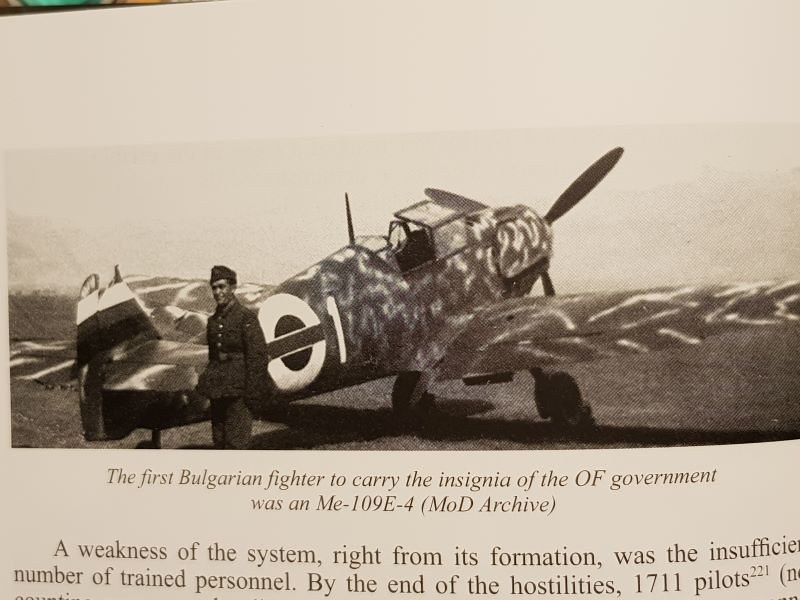The image, likely sourced from a vintage publication such as a history book or an old newspaper, features a black and white photograph in landscape orientation. The top two-thirds of the image showcase a vintage warplane, specifically an ME-109E-4, adorned with camouflage paint and white lettering on its side. The plane’s cockpit, which has been designed to allow the glass canopy to be removed, is visible in the image. Standing near the tail end of the aircraft is a man dressed in a military uniform. The caption under the photograph reads, "The first Bulgarian fighter to carry the insignia of the OF government was an ME-109E-4 (MOD archive)." Below this, the text continues, "A weakness of the system, right from its formation, was the insufficient number of trained personnel. By the end of the hostilities, 1,711 pilots…" The rest of the text is cut off, and there appears to be a reference marked as “221.” The overall appearance of the image and text suggests a historical context, emphasizing its informative nature regarding Bulgarian aviation history.